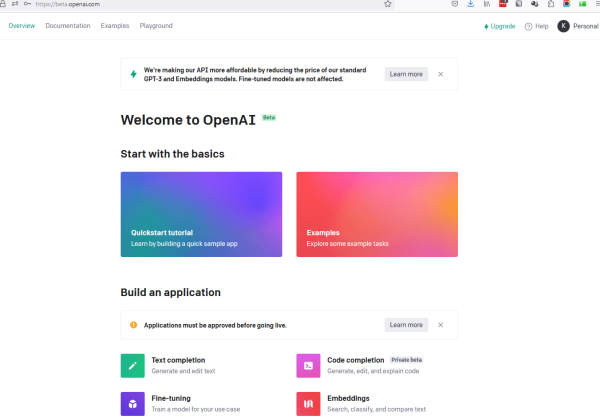Screenshot of the OpenAI Beta Website on a Computer Screen

The image captures a screenshot of the OpenAI website as viewed from a computer screen. At the very top, there is a faint gray bar displaying the URL: "http://beta.openai.com." The main body of the webpage has a white background, providing a clean and minimalistic appearance. Centrally, two large rectangles catch the eye—the first rectangle blends shades of purple and green, while the second rectangle features a gradient of pink transitioning through deep to light orange. Above these vibrant rectangles, large black text prominently displays "Welcome to OpenAI," followed by a smaller, but still noticeable, "Start with the basics." Beneath the two colored rectangles, additional black text guides the viewer with the words "Build an application."